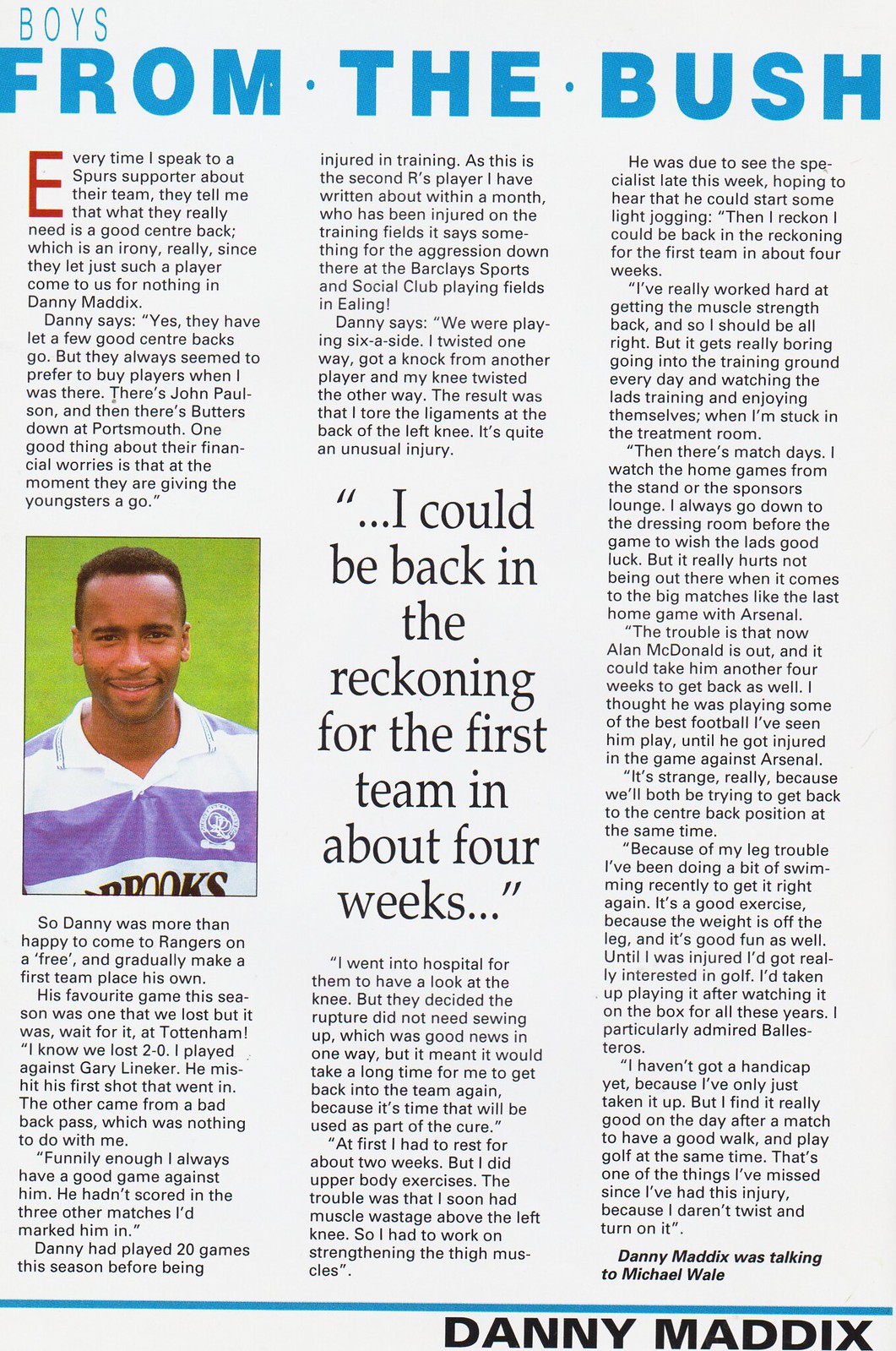This image appears to be a scan from an interview page out of a magazine, featuring Danny Maddox. The top of the page prominently displays the title "Boys from the Bush" in large blue letters. The layout includes three columns, with an image of Danny Maddox, a black man in a purple and white shirt, situated in the middle left section. The text contains several paragraphs detailing a conversation between Danny Maddox and the interviewer, Michael Whale. Notably, there's a highlighted quote in the center of the page that reads, "I could be back in the reckoning for the first team in about four years." The interview starts with an observation about the Spurs' need for a good center back, ironically mentioning that they let Maddox go to his current team for nothing. Throughout the article, Maddox discusses the team's inclination to purchase established players over nurturing young talent. At the bottom of the page, it is reiterated that "Danny Maddox was talking to Michael Whale," with a final dark-lettered mention of his name beneath a blue line stretching across the page.